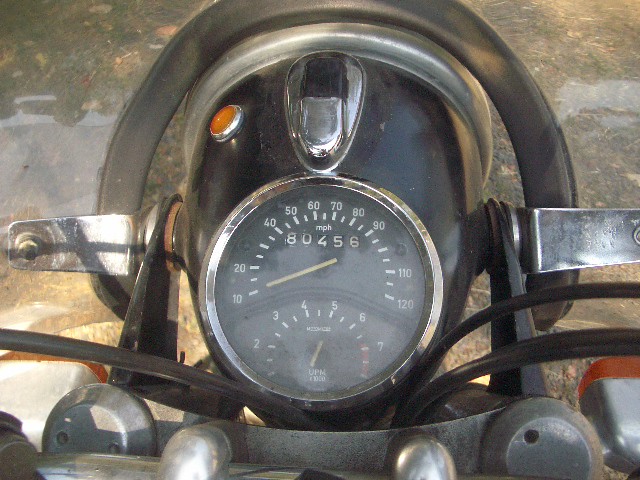A top-down, point-of-view photograph captures the speedometer and odometer of a vintage, tarnished motorcycle, highlighting its aged character. The metal components and finishes exhibit significant tarnish, emphasizing its old age. The motorcycle itself is black, matching the black background of the well-lit speedometer and odometer dials. White text marks the speedometer, while yellow needles indicate the speed; the odometer reads a total mileage of 80,456. The photograph, taken outdoors on a sunny day, reveals a slight ground reflection in the background, suggesting a recent rain. Several wires emerge from beneath the centrally positioned speedometer, adding to the motorcycle's weathered charm. The moderate quality of the image still effectively conveys the aged yet robust nature of this classic motorcycle.